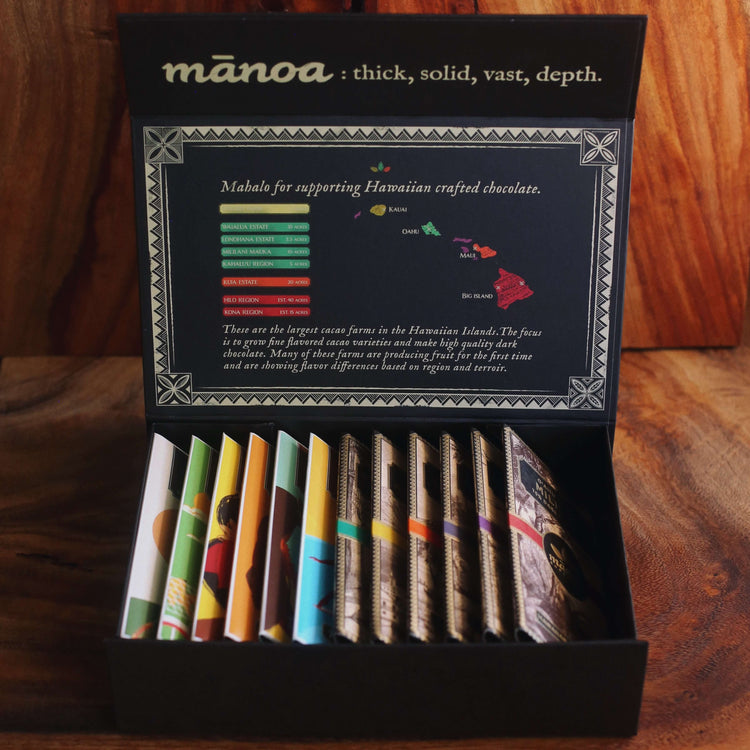The image presents an open black box resting on a brown wooden surface, with visible wood grain rings. On the inside of the box’s lid, the word “Manoa” is prominently displayed, described as "thick, solid, vast depth." Surrounding this area is a white border featuring symbols in each corner. Below this, a color-coded map of Hawaii shows the islands highlighted in various colors. The text on the lid expresses gratitude: "Mahalo for supporting Hawaiian crafted chocolate," and continues to explain that these are the largest cacao farms in the Hawaiian Islands. The focus is on cultivating fine-flavored cacao varieties to produce high-quality dark chocolate. Notably, many of these farms are producing fruit for the first time and are starting to reveal flavor differences based on their specific regions and terroir. Within the box itself, there are multiple chocolate bars neatly arranged, showcasing a variety of colors such as yellow, green, orange, and red. Additionally, six bars on the right are predominantly white with colored stripes in hues like teal, yellow, orange, light purple, violet, and another orange.